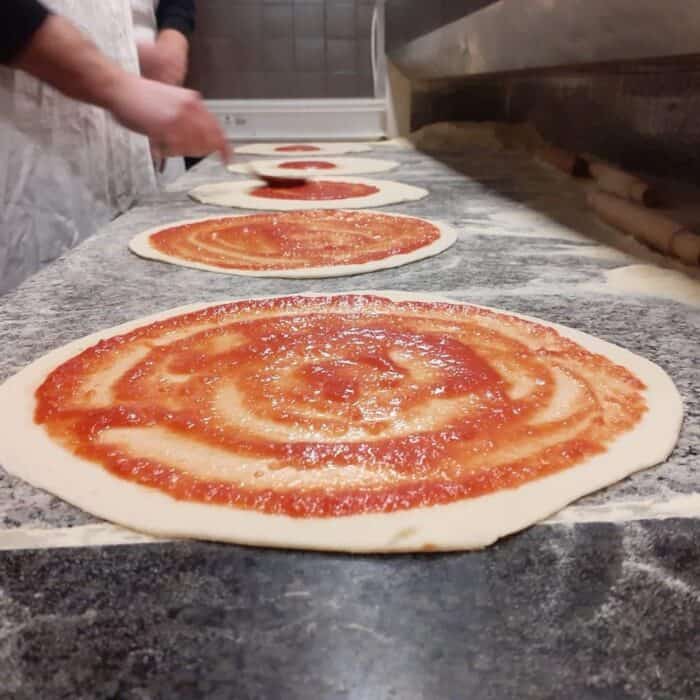A meticulous scene unfolds in a bustling pizzeria kitchen, where a dedicated pizza maker is in the process of crafting thin-crust pizzas. The marble countertop stretches out before him, peppered with fine cornmeal and hosting a lineup of five pizzas. Each pizza is arranged in a sequential row, drawing the eye from the foreground to the distance, creating a sense of depth. The first two pizzas are already adorned with a smooth layer of tomato sauce, indicative of the early stages of preparation. The third pizza is in mid-process; the pizza maker, whose visage is partially visible from the chest to the waist, spreads the sauce with skillful precision using a spoon. The fourth and fifth pizzas await their turn, with dollops of sauce in the center, yet to be evenly distributed. To the right of this orchestrated culinary activity, a pizza oven stands ready to receive the finished creations. The pizza maker, a Caucasian individual garbed in a white apron, focuses intently on his task, his arms and hands moving with practiced expertise. This snapshot captures the heart of pizzeria operations, showcasing the artistry and diligence involved in preparing delectable pizzas.